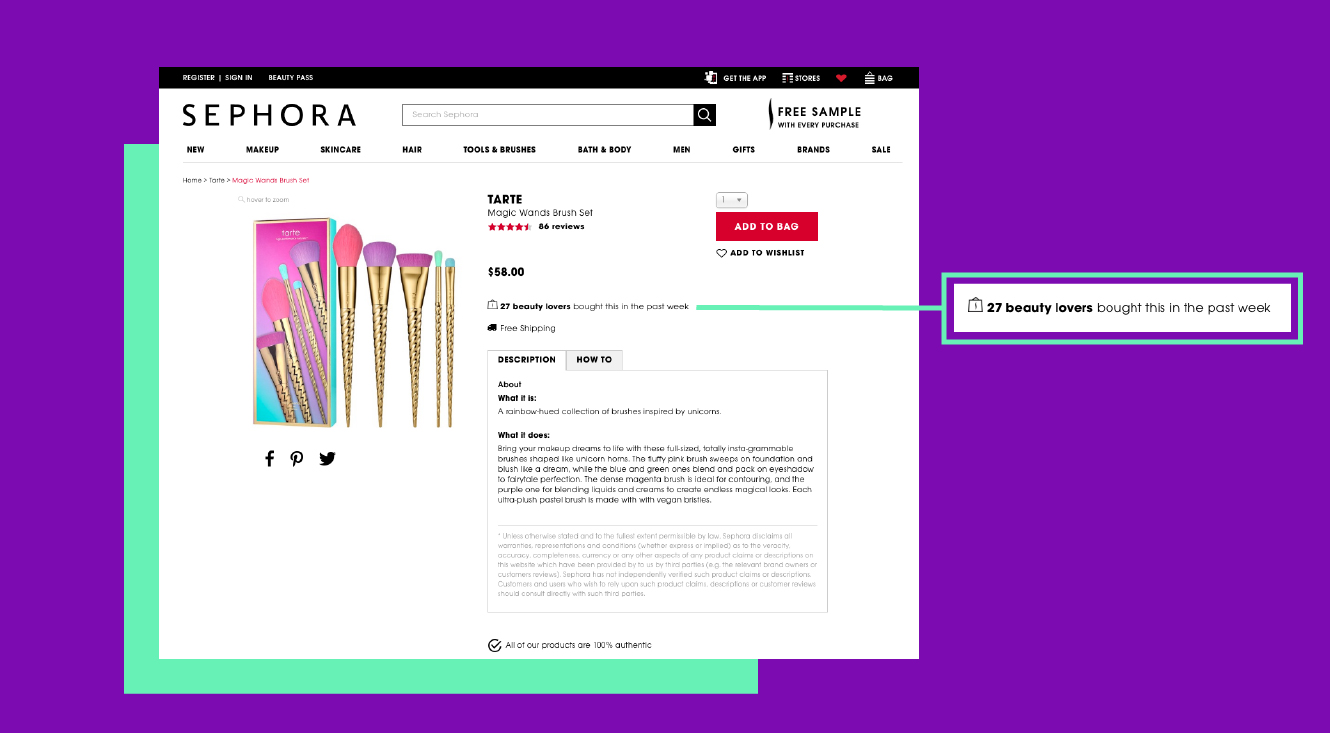The image features a visually appealing purplish-blue background. In the lower-left corner, a teal square overlaps partially with a white square. The top portion of the white square has a black background containing white text. On the left side, the text reads "Register/Sign In." Adjacent to this, another section displays "Beauty Pass," followed by a blank space. 

To the right, an illustration of a phone appears with the text "Get the App," followed by icons and labels such as "Stores," a red heart, and "Bag." Above this, there's a black text on white background that reads "Sephora," alongside a white search bar. Further to the right in black text, it mentions "Free Sample," although the text is partially cut off.

Below this section, ten clickable categories are displayed in black text. The text is difficult to read, but the first category appears to say "New," and the last one on the far right reads "Sale."

Centered below these elements is a gold-colored brush set consisting of five makeup brushes: three large and two smaller ones. The bristles are colored variably, with pink on the leftmost brush, proceeding to light purple, dark purple, creamy white, and ending with a bluish hue on the smallest brush. 

To the right of the brush set, under the brand name "Tarte," the price is listed as $58. An "Add to Bag" option is also provided. The overall composition is vibrant and visually engaging, marking it as a sophisticated promotional image.